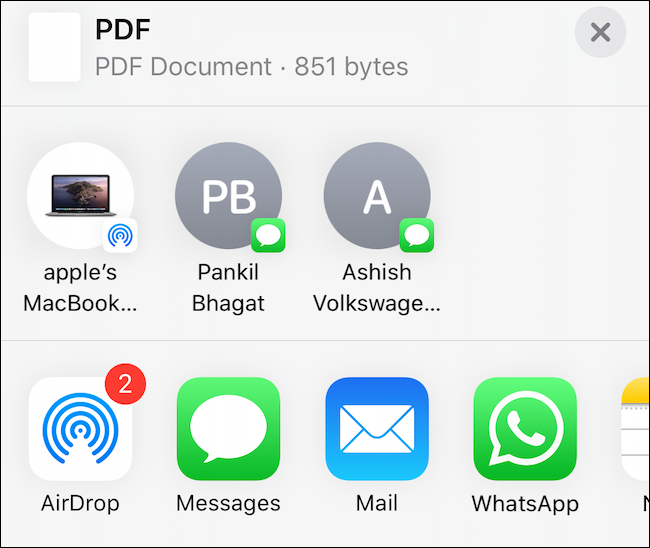The image depicts a MacBook screen featuring a white square icon labeled "PDF" representing a PDF document of 851 bytes. On the top right corner of this icon, there is a gray circle. The background of the screen is gray. Additionally, there are various icons and elements displayed, including:

- A blue square at the middle-bottom of the image, which is accompanied by a speech bubble icon.
- A green square with a speech bubble containing a handset inside, indicating the WhatsApp application.
- An icon resembling a notepad which symbolizes the Notes application.

Other details include:
- Three circles and five squares scattered throughout the image.

This detailed caption comprehensively describes the elements and layout featured on the MacBook screen in the image.